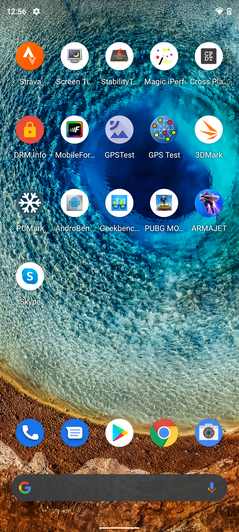A screenshot captures the home screen of an Android mobile phone, evident by its distinct layout characteristic of non-Apple devices. The screen's background features a vibrant tropical theme with clear, crystal blue water meeting an orangish-brown sandy shoreline, evoking a serene beach setting. 

At the top left corner, the time is displayed as 12:56, although it is unclear whether it is AM or PM. Adjacent to the time, icons indicate the Wi-Fi signal strength and the phone's battery level.

The home screen is populated with a variety of application icons. Notable among these are Strava, 3DMark, two GPS test applications, PubG, Skype, the Google suite, and the Microsoft Store. Some icons appear partially cut off, making the identification of certain apps challenging. Other discernible app names include Screen Time, Stability, and Magic. The structured yet bustling arrangement of applications reflects a well-utilized and personalized device.